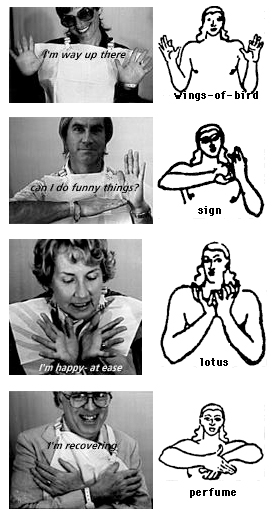This detailed black-and-white image features two vertical columns, juxtaposing four pairs of photographs and illustrations. The left column exhibits four black-and-white thumbnail photographs, while the right column presents corresponding line drawings depicting similar hand signs from sign language.

At the top left, a photograph shows a woman holding up a shirt that says "I'm way up there," accompanied by a stick figure on the right with both hands raised, labeled "Wings of a Bird." Below this, another black-and-white photo features a man making the sign with his right hand flat against the bottom of his left palm, captioned "Can I do funny things?" with a corresponding drawing titled "Sign."

The third row presents a black-and-white photo of a woman with her hands open in front of her, the heels of her hands touching while her fingers are outstretched, stating "I'm happy and at ease." On the right, a drawing mirrors her hand gesture, labeled "Lotus." 

Finally, at the bottom left, a man wearing glasses smiles with his arms crossed, under the caption "I'm recovering." The adjacent drawing replicates his gesture and is labeled "Perfume." Each pair illustrates how specific sign language gestures are represented both photographically and through line art, providing a visual comparison between real-life hand signs and their drawn counterparts.